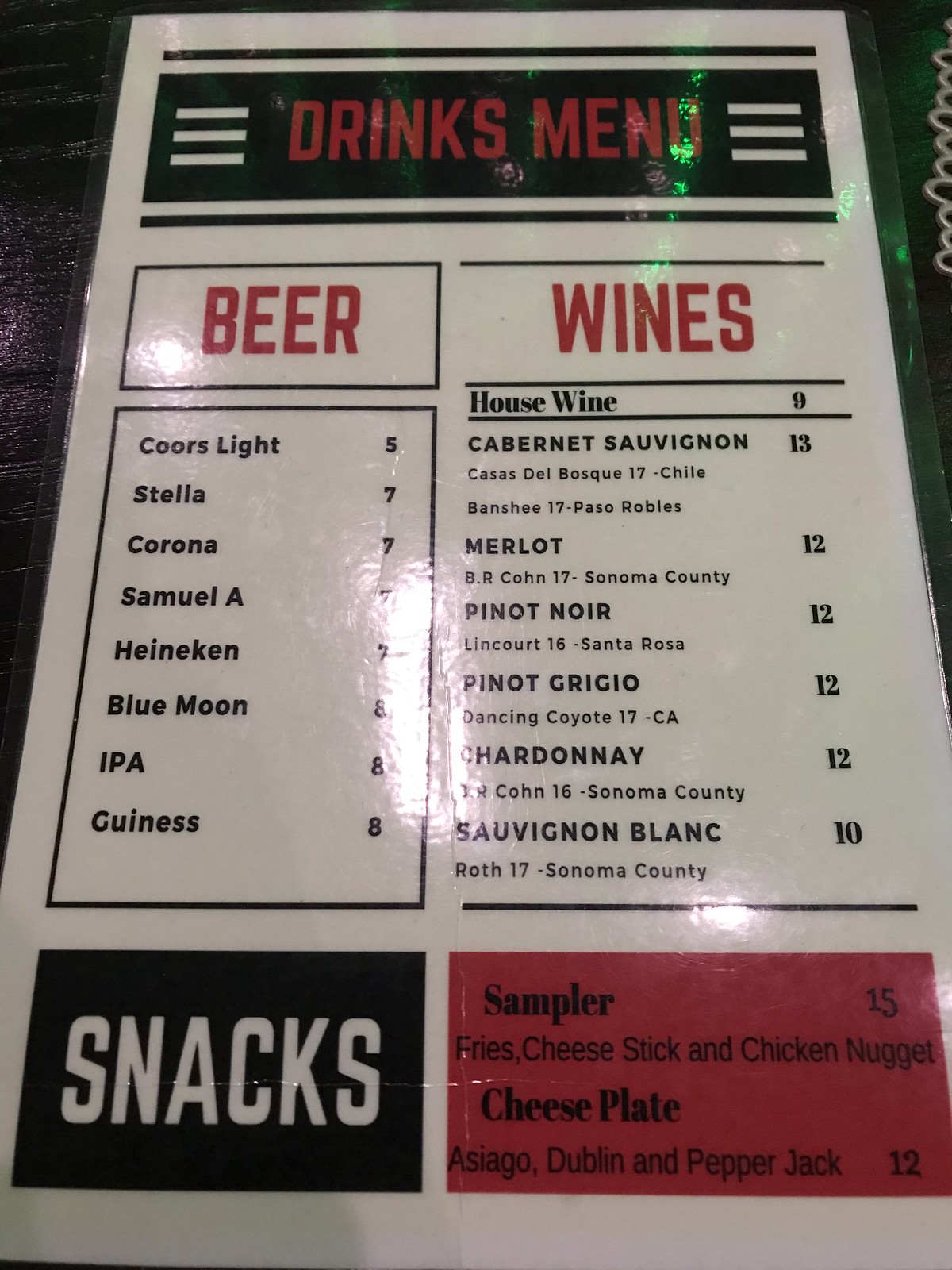This image features a neatly organized, portrait-style drink and snack menu from a restaurant, presented in a monochromatic palette of black, white, and red. The design utilizes bold, blocky letters for section headers and a mix of Impact and Times New Roman fonts for item descriptions, creating a visually striking and easy-to-read layout. 

At the top, the header reads "Drinks Menu." Below it, the menu is divided into two sections, each occupying its own column: "Beer" on the left and "Wines" on the right.

In the "Beer" section, the offerings are listed along with their prices:
- Coors: $5
- Stella: $7
- Corona: $7
- Samuel A: $7
- Heineken: $7
- Blue Moon: $8
- IPA: $8
- Guinness: $8

The "Wines" section lists the options and their prices, along with details about the origin, year of the grapes, and the vineyard:
- House Wine: $9
- Cabernet Sauvignon: $13
  - Casas del Bosque, 2017, Chile
  - Banshee, 2017, Paso Robles
  - [Further details follow in similar format]

At the bottom of the menu, the "Snacks" section features:
- Sampler Platter: $15
  - Includes fries, cheese sticks, and chicken nuggets
- Cheese Plate: $12
  - Includes Asiago, Dublin, and Pepper Jack cheeses

This detailed and structured menu ensures that patrons can easily navigate their beverage and snack options while appreciating the clarity and simplicity of the design.